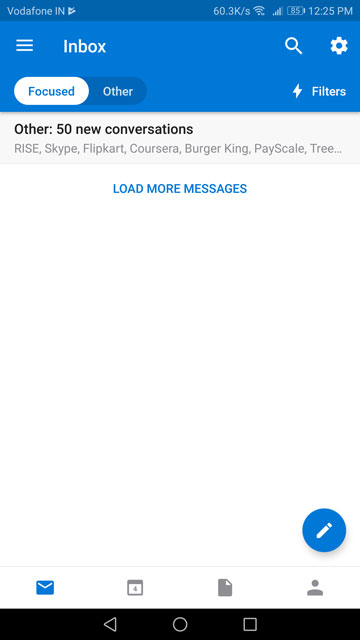This screenshot captures a mail application on an Android device. The telltale Android navigation icons at the bottom of the screen (back arrow, circle home button, and square overview button) confirm the device type. The app features a blue and white theme, with a prominent blue header at the top. 

In the blue header, a hamburger menu button is on the upper left corner, adjacent to the word "Inbox" written in white text. On the right side of the header, there are a magnifying glass icon for search and a gear icon for settings. Below the header, there are two tabs: "Focused" and "Other." Currently, "Focused" is selected, highlighted in white, while "Other" is in dark blue. 

Underneath the tabs, there's a section that indicates "Other, 50 new conversations," with a list of senders including Rise, Skype, Flipkart, Coursera, Burger King, and PayScale. At the bottom of this section, there's an option to "Load more messages" in blue text. 

Additionally, in the bottom-right corner of the screen, there is a blue circular button with a pencil icon, indicating the option to create a new message.